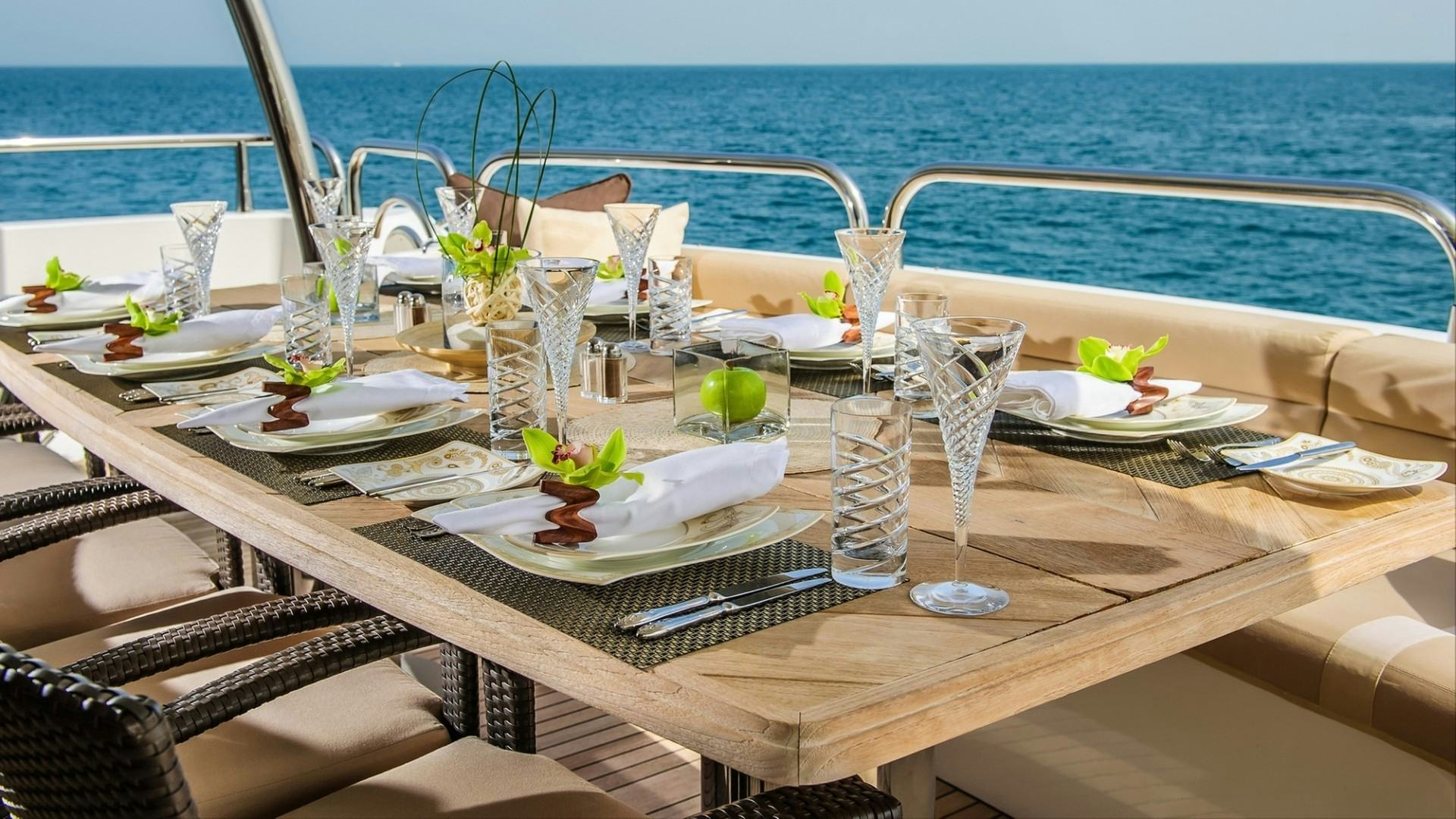This photograph captures a meticulously set dining table on a yacht gliding over clear ocean waters under a sunny, blue sky. The table, which appears to be made of wood, is elegantly arranged with eight matching place settings. Each setting includes a plate adorned with a decorative bundle of napkins held by a small wooden spiral and a couple of leaves. To the right of each plate are two butter knives, while two forks are placed to the left. Between each main plate setting, there is a small square plate also accompanied by a butter knife.

In front of each plate, there are two types of glasses: a wine goblet with a crisscross design and a shorter round glass with a spiral net pattern. The centerpiece of the table features a green apple enclosed in a glass box, alongside a pepper shaker, a salt shaker, and a wooden bowl containing a white substance. 

The dining area is flanked by tan cushion chairs with wicker-type armrests and backs on three sides, while the right side of the table offers a long bench with tan and white cushioning. Chrome railings of the yacht are visible behind the table, framed against the backdrop of the expansive, clear waters and the shadow they cast, indicative of a beautiful, tranquil daytime setting.